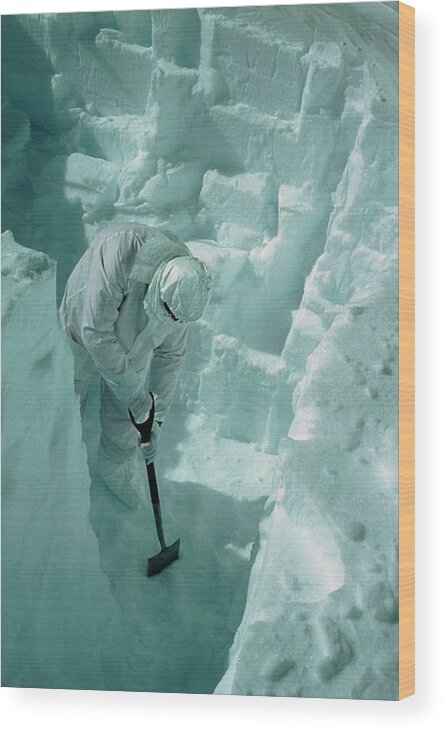The image depicts a canvas print showcasing a man on a glacier, engaged in intense digging with a rusted shovel. Dressed in an all-white outfit resembling a hazmat suit, the man is slouched over, persistently shoveling through the snow and ice. His attire includes a hood with slits for his eyes, leaving the rest of his face obscured. The snow around him has been significantly displaced, indicating extensive excavation. The print itself is marked with lines suggesting it has been enlarged beyond its optimal resolution. A shadow cast by the man is visible in the snow, adding depth to the scene. The overall atmosphere conveys a sense of struggle, as if the man might be attempting to tunnel out or possibly rescue someone trapped beneath the ice. The edges of the image are light brown, contributing to its canvas-like texture.